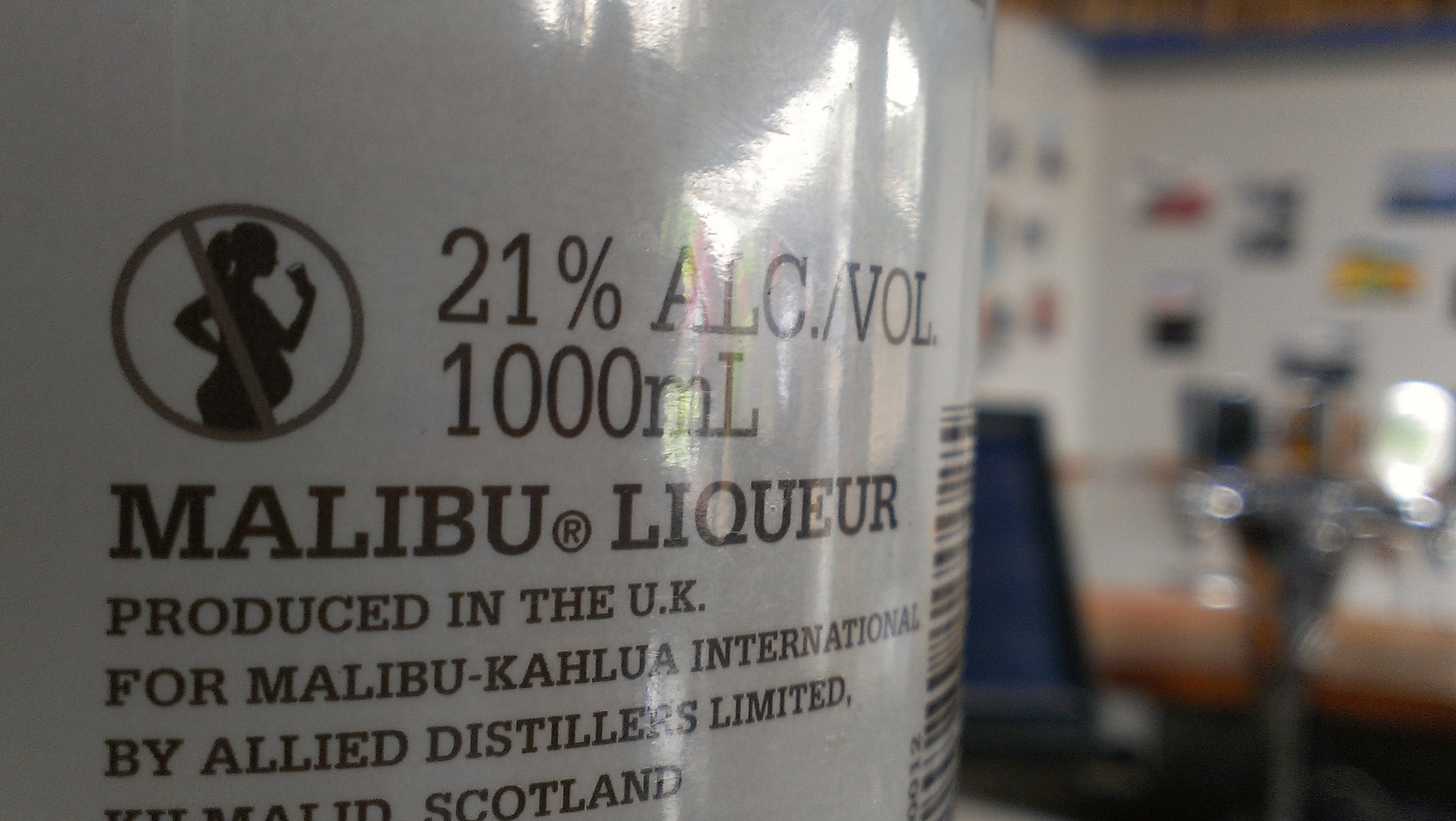This close-up image captures a portion of a shiny white bottle label, specifically highlighting critical information and symbols. On the upper left side of the label, an icon depicts a pregnant woman drinking with a circle and a line through it, clearly indicating that the alcohol is not safe to consume during pregnancy. The label text prominently states "21% ALC / VOL, 1000 milliliters" in brown lettering. Below this, it reads "Malibu® Liqueur produced in the UK for Malibu Kahlua International by Allied Distillers Limited," with a mention of Scotland, though slightly obscured. You can also see the edge of a barcode as the label curves around the bottle. The background is a blurry interior, possibly a bar, lounge, or club room, featuring a table with chairs and some items on the walls.